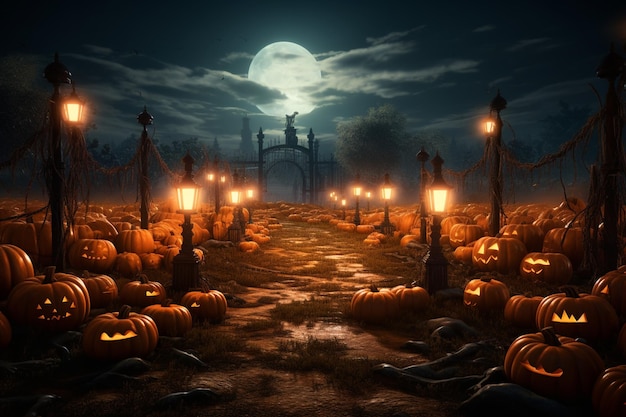This digitally-rendered, Halloween-themed image captures a spooky night scene dominated by a large, glowing full moon partially veiled by wispy clouds. The focal point is a winding pathway that bisects the composition, stretching towards an intricate, ornate metal gate at the far end, which is faintly visible due to its distant placement. Flanking both sides of the path are hundreds of jack-o'-lanterns, some traditionally carved with triangle eyes, noses, and jagged mouths, while others feature simpler cutouts. The pumpkins are arranged within what appears to be a pumpkin patch, adding to the eerie atmosphere. Illuminating the pathway are various street lamps and lanterns, both large and small, casting a ghostly glow that accentuates the Halloween ambiance. In the background, silhouettes of trees and unidentified buildings emerge, partially obscured by the dense arrangement of pumpkins and the soft, diffused light. The scene is intricately detailed, yet certain elements exhibit subtle imperfections, suggesting an AI-generated origin. This haunting visual could easily transport viewers into a surreal, nightmarish Halloween landscape.